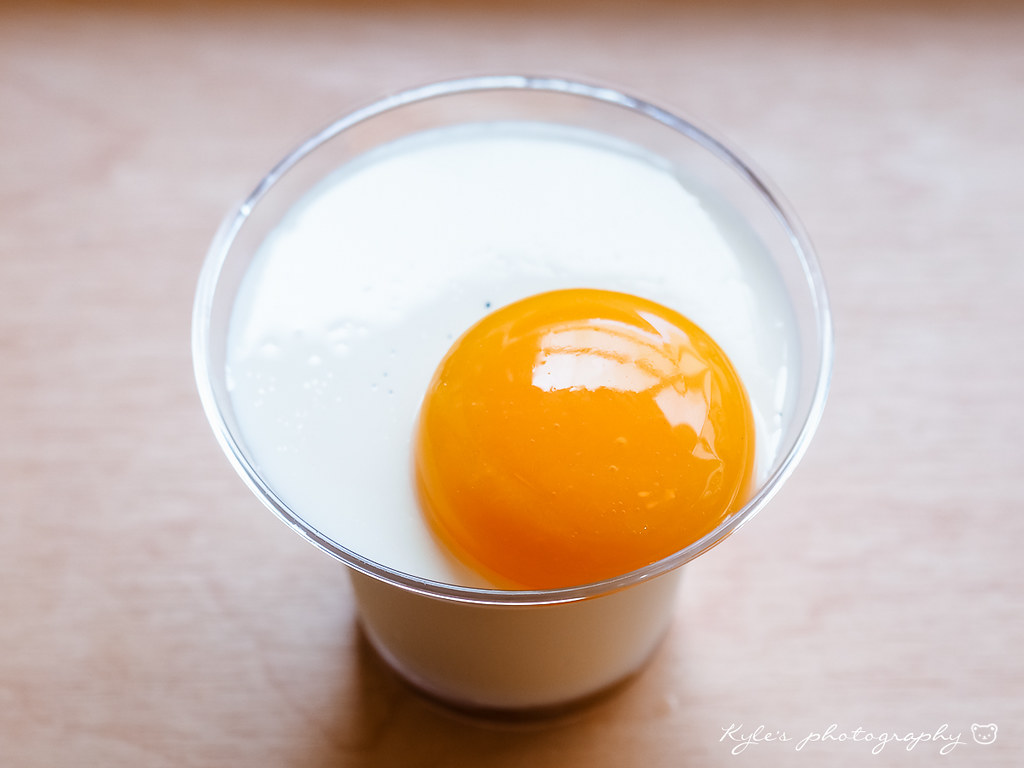The image depicts a clear glass sitting on a light beige surface, perhaps a countertop or a wooden table. Inside the glass is an egg yolk nestled within a white, semi-solid or liquid substance, possibly milk. There's some ambiguity regarding the consistency and exact nature of the white content inside the glass. A shadow is cast by the glass on the surface below. The photograph is taken from above, at an approximate angle of 30-40 degrees. The wide rim of the glass is notable in contrast to its body. In the bottom right corner of the image, there is a barely readable inscription in thin white print that reads "Kylie Photography," alongside a small bear illustration or smiley face, both set against the light surface, making it difficult to discern clearly.